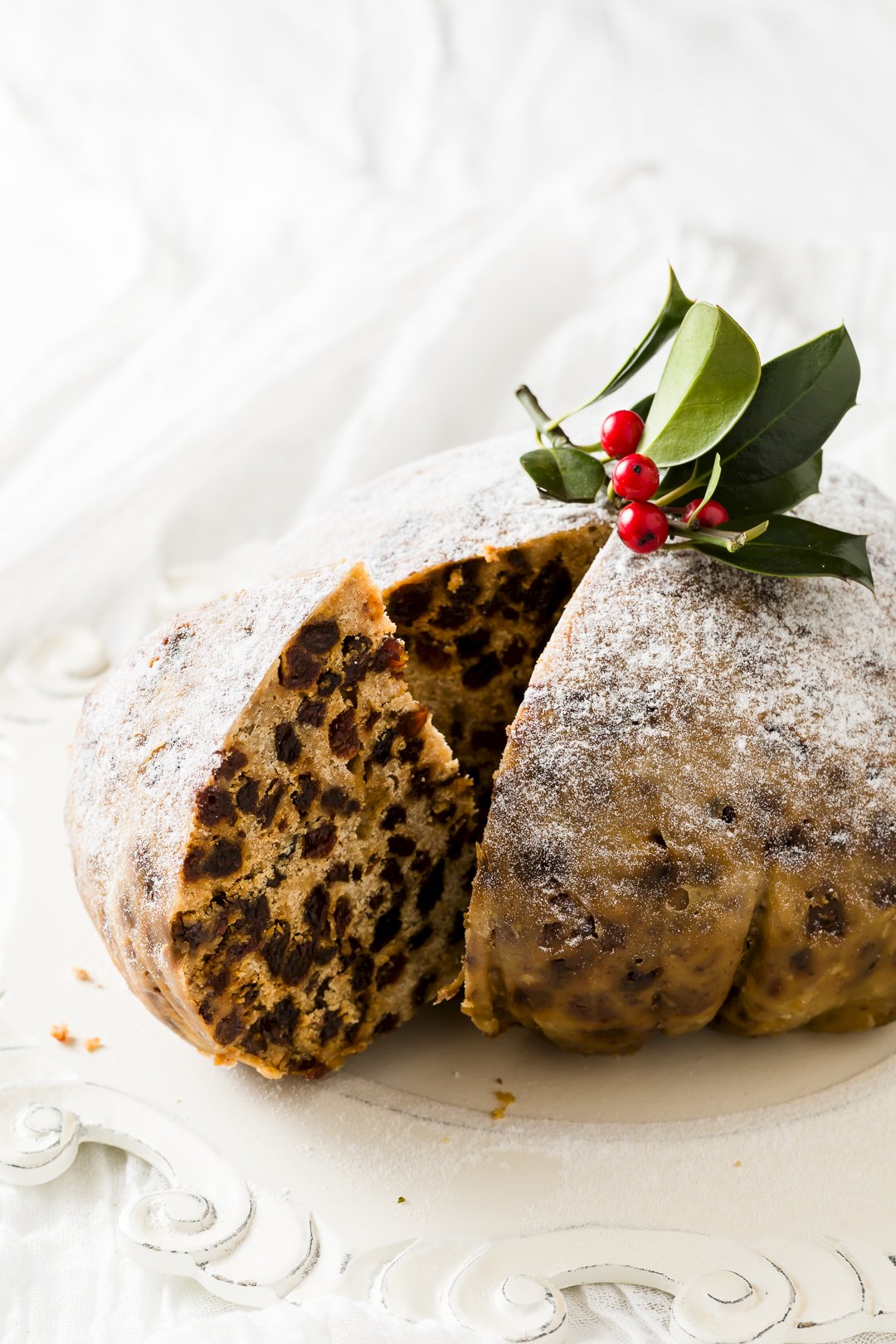This photograph depicts a round, homemade dessert bread with an oblate shape, featuring a light brown exterior sprinkled with a fine dusting of powdered sugar. The loaf is seated on a rustic wooden serving platter with worn, filigree edging, all set against a stark white, rippled fabric background. A thick, triangular wedge has been cut from the loaf, revealing a cake-like interior dotted with what appears to be raisins, dates, or possibly melted chocolate chips. Garnished on top with a festive sprig of holly and vivid red berries, the bread exudes a homely charm, lending itself well to a bright, naturally lit indoor setting. The bread's enticing presentation suggests it might be featured on a website for culinary enthusiasts or product advertisement.